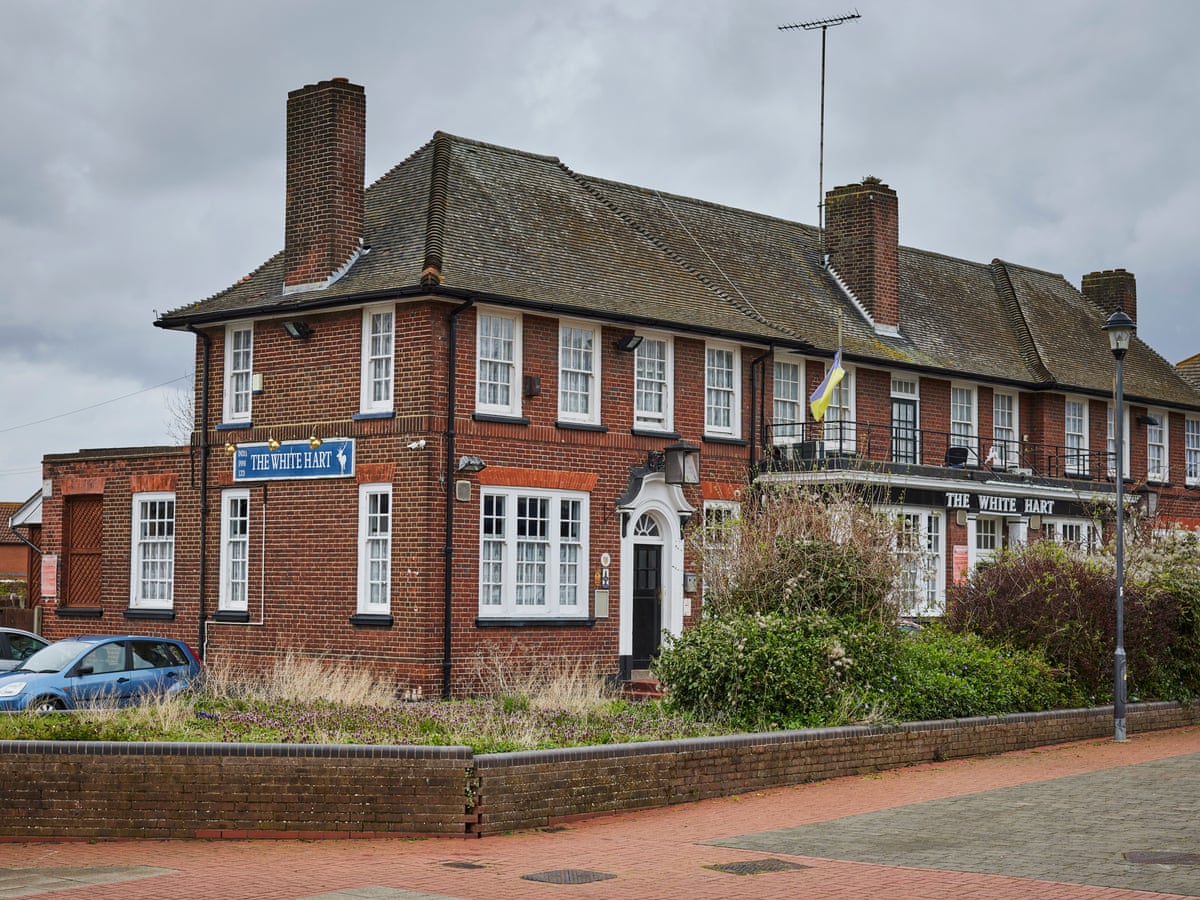This is a color photograph of a large, two-story building constructed from red and brown bricks, complemented by a sloping brown roof. Prominently featured is a red brick chimney on which a TV antenna is mounted. On the side of the building, a sign reads "Heart" (stylized as "H-A-R-T") alongside a silhouetted drawing of a white heart, with the same "H-A-R-T" and heart graphic repeated on a black overhang above a black doorway at the front.

The facade of the building showcases numerous windows, lending an air of openness and inviting natural light. A distinguishing feature is a flying purple and yellow flag attached to a balcony. To the far left, several vehicles are parked, adding context to the building’s use and suggesting it might be a place of business or community gathering.

The sidewalk in front of the building is paved with matching brown and red bricks, creating a unified aesthetic with the building's exterior. Under an overcast sky, the ambiance is subdued with gray clouds looming, yet the tall streetlight standing nearby promises illumination when needed.